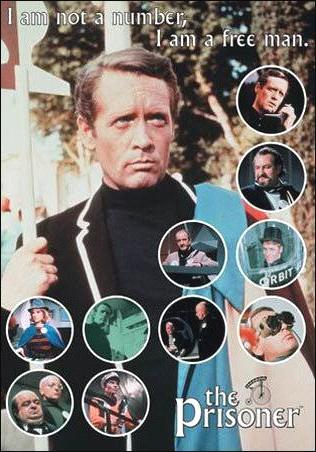The poster from the movie *The Prisoner* prominently features a slogan in white text across the top that reads, "I am not a number, I am a free man." Central to the poster is an image of a white man with medium-length brown hair, dressed in a black turtleneck and a black suit jacket with a white-bordered lapel. His left hand holds a stick-like object. Surrounding him are multiple circular thumbnails, each depicting different characters or scenes from the movie. The color palette includes beige, light blues, greens, reds, blacks, grays, tree bark brown, tree green, and orange. At the bottom right corner of the poster, the movie title "The Prisoner" is written in white text with a black outline. The overall style suggests the poster might be from the 60s or early 70s.